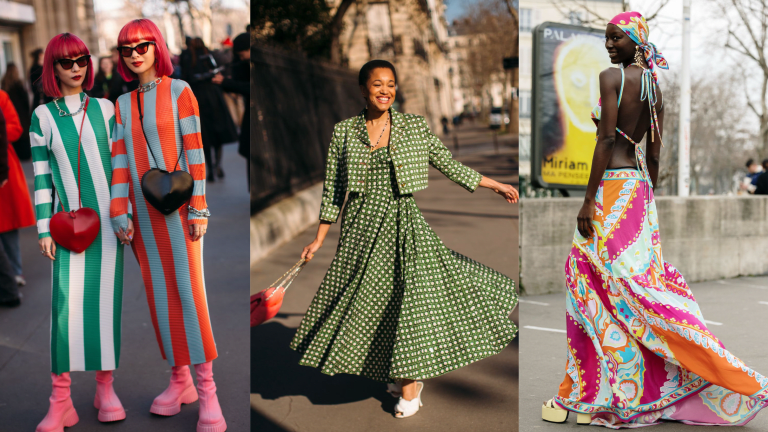The image is a horizontal collage of three different photos featuring stylish women, likely models, in vibrant and trendy outfits. On the left, two women with shoulder-length pink hair are seen standing on a bustling street. Both are wearing sunglasses and striped dresses—one in green and white with a red heart-shaped purse, and the other in gray, blue, and orange with a black heart-shaped purse. They are also both wearing eye-catching pink boots. The central photo showcases a smiling woman, casually walking down a street in a green dress adorned with white polka dots. She has short black hair and is accessorized with a green jacket, white shoes, and an orange handbag. In the rightmost photo, a black woman is posing with a colorful headscarf, vibrant backless top, and long skirt in front of a sidewalk and a small stone wall. She appears to be wearing high-heeled sandals and is looking back at the camera, with distant onlookers and a poster in the backdrop. The collage emits a lively and diverse fashion statement with a mix of playful colors such as pinks, greens, oranges, blues, and various tones of beige and brown. These images are connected by their vibrant fashion choices and dynamic street settings.